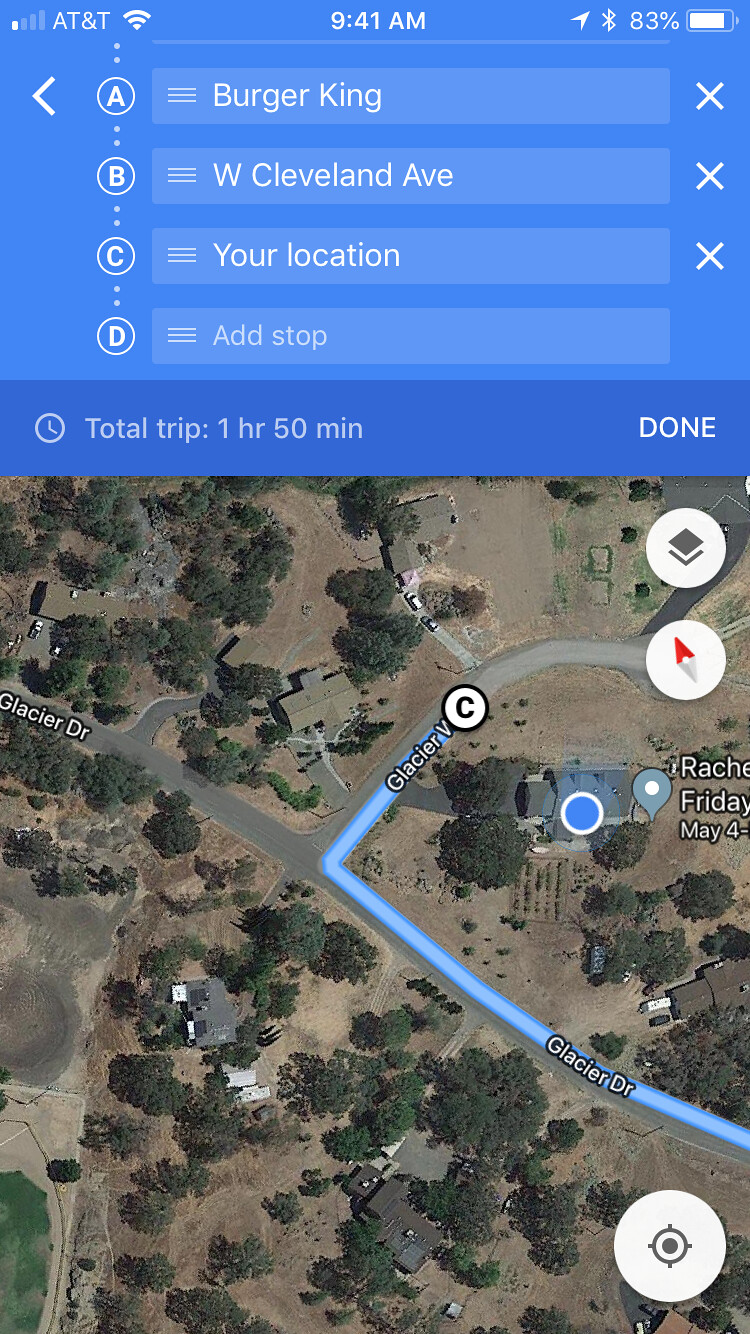This is a detailed screenshot taken from a navigation app, likely Google Maps. At the top of the image, the status bar displays the Wi-Fi signal strength, indicating the device is connected to a network, and the mobile carrier is AT&T. The current time is 9:41 AM, shown centrally on the status bar. On the right end of the status bar, the Bluetooth symbol is visible, alongside an indication that the phone's battery is at 83%.

Within the app interface, the map route includes multiple stops: 'A' is designated as Burger King, 'B' is West Cleveland Avenue, 'C' marks the current location of the user, and 'D' is an available slot for adding an additional stop. The total estimated trip duration is 1 hour and 15 minutes. 

A significant portion of the screenshot is occupied by the map itself. Notable streets visible include Glacier Drive and Glacier View, although part of the latter's name is cut off and it is likely intended to read Glacier View Drive or similar. The map offers a visual representation of the route alongside these geographic details.